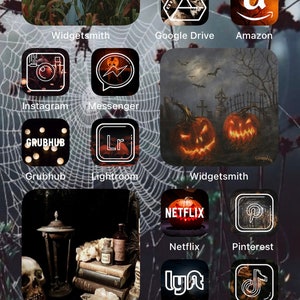This image is a detailed screenshot of a small mobile or tablet device, most likely running an Android operating system, given the layout and positioning of the icons. The device screen features a spooky Halloween theme. 

The background image showcases an intricate spider web with a spider perched on it, setting a creepy tone. Overlaid on the background are additional themed images provided by the app "Widget Smith." In the top left corner, a "Widget Smith" widget partially obscures an image. To its right, another "Widget Smith" widget vividly displays two eerie jack-o'-lanterns set against a cemetery backdrop, complete with bats, a cloudy night sky, and a glowing moon. The bottom left corner features a morbid setup with a skull, an urn, several books, and what seems to be a poison bottle.

The user's app icons contribute to the spooky aesthetic with a predominantly black theme adorned with tiny jack-o'-lanterns and cobwebs. The visible apps, ordered from left to right, include:
- Google Drive
- Amazon
- Instagram
- Messenger
- Grubhub
- Lightroom
- Netflix
- Pinterest
- Lyft
- TikTok

Overall, the screenshot artistically captures the personalized Halloween-inspired layout on the user's device, highlighting their affection for the spooky season.